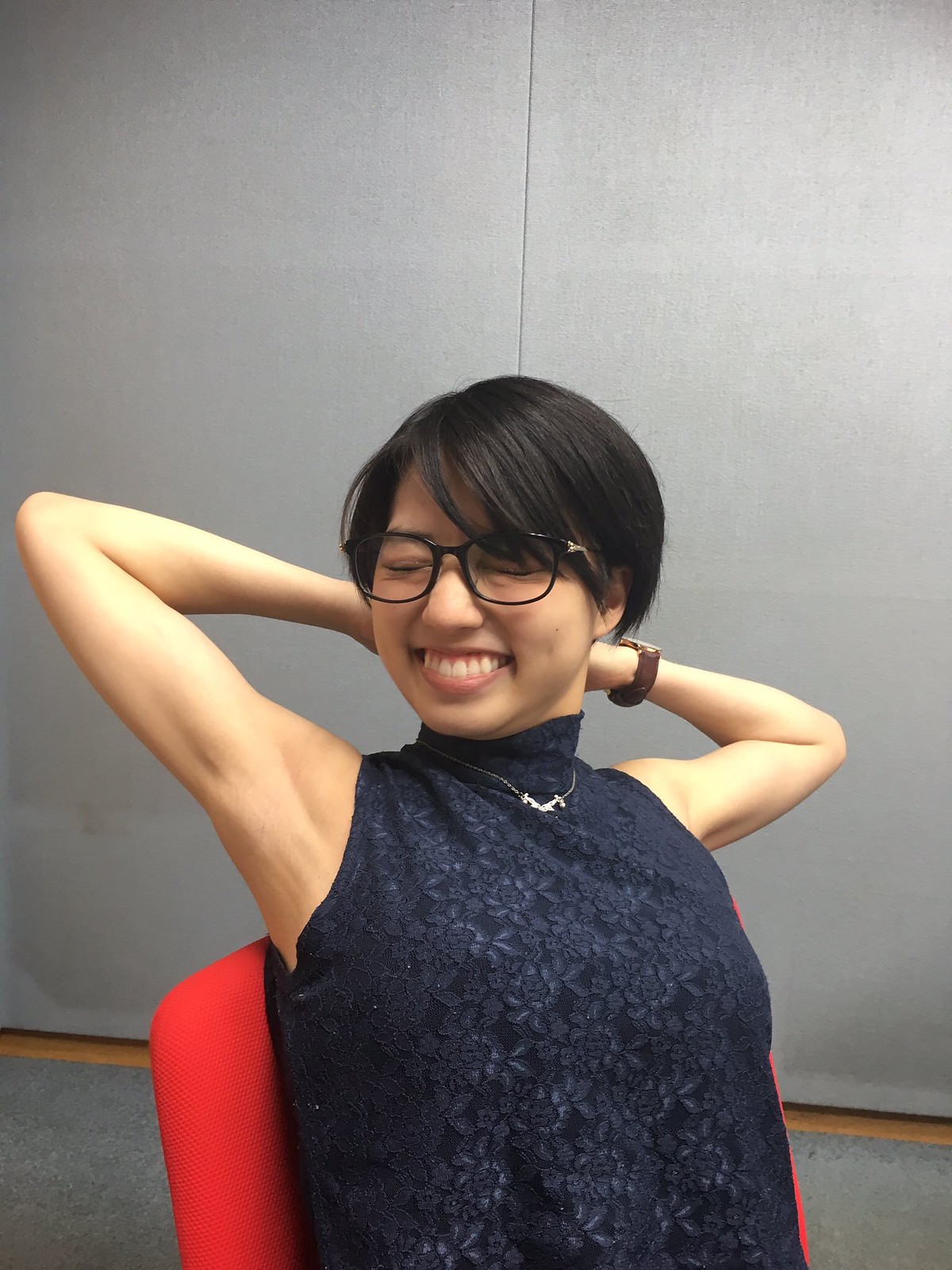In this indoor photo, a woman, likely of Asian descent, is seated in a stationary, bright red office chair. She is stretching with both arms placed behind her head, her elbows bent, and her eyes closed in a serene smile. The woman is clad in a black sleeveless blouse featuring a turtleneck and accessorized with a delicate silver necklace. On her wrist, she wears a brown wristwatch. She has short black hair that just slightly passes her ears and dons black glasses. The background showcases a gray wall with a noticeable crease where two panels meet, along with a wooden trim at the base and a gray floor that matches the wall. The overall ambiance captures her enjoying a moment of relaxation.